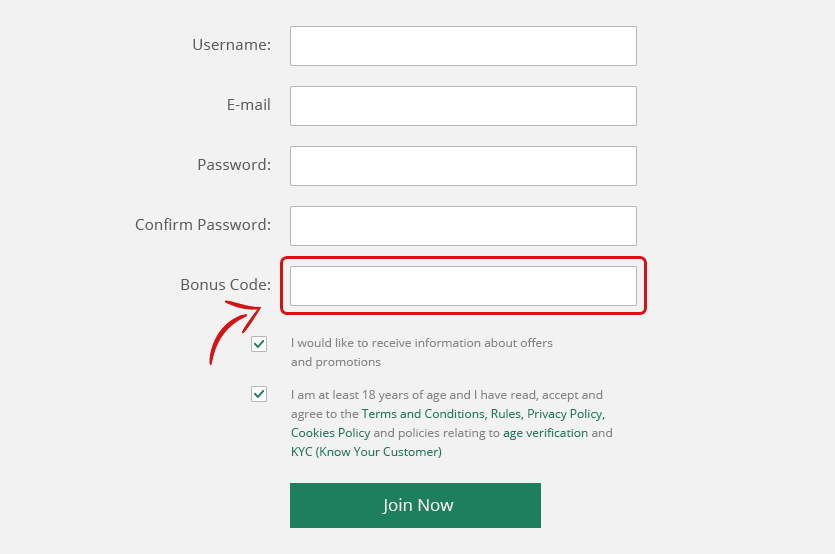Caption: 

The image showcases a detailed, color sign-in page with a whitish-pink background. At the top of the page, there is a textbox labeled "Username," where users are prompted to enter their username. Directly below this textbox, fields for "Email" and "Password" are present, followed by another field to confirm the password. 

Additionally, a distinct section labeled "Bonus Code" is highlighted with a red arrow and circled for emphasis. Beneath the Bonus Code section, there are two checkboxes, each marked with a green checkmark. The first checkbox is accompanied by the text, "I would like to receive information about offers and promotions." The second checkbox, also marked, states, "I am at least 18 years of age; I have read, accepted, and agreed to the terms and conditions, rules, privacy policy, cookies policy, and policies relating to age verification and KYC (Know Your Customer)."

At the bottom of the page, a prominent green "Join Now" button invites users to complete their registration process.